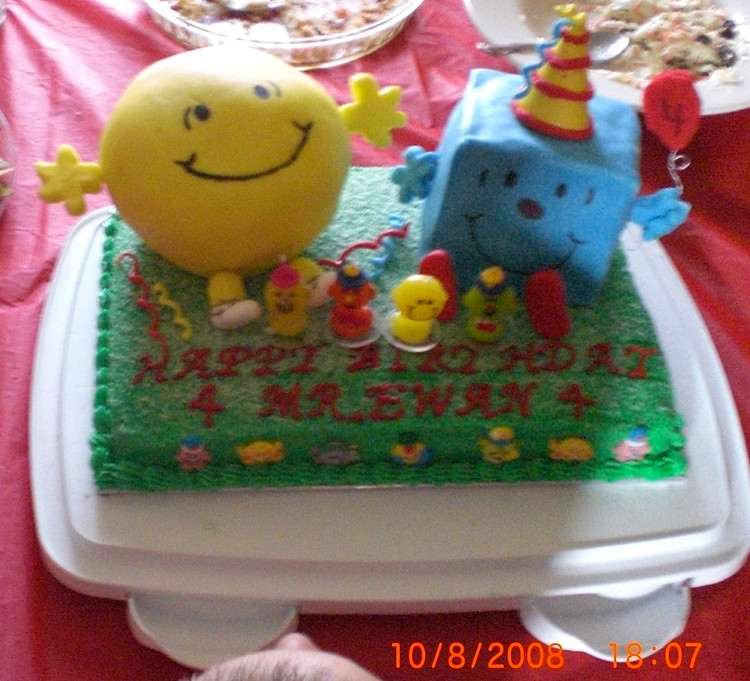This photograph captures an overhead view of a festive birthday scene. Centered on a table draped with a pink tablecloth, adorned with a few wrinkles in the top left and right sides, is a birthday cake. The cake, accented with green icing, bears the red-iced inscription, "Happy Birthday Mr. Ewan." The cake features two prominent cartoon-like characters: a large, round, yellow figure with outstretched hands, white feet, and a big smile, and a smaller, square blue figure with a party hat adorned with alternating red and yellow stripes. This square character holds a red balloon with the number "4" in white. Around them are four smaller characters sitting on the cake in front of the larger figures, adding to the whimsical decoration. Along the bottom of the cake, in red icing, the date "10/8/2008" and the time "18:07" are inscribed, marking the special occasion. In the peripheral corners of the image, partially visible, are additional items on the table: a plastic container with some candy or food in it at the top left and a plate with a spoon in the top right, hinting at the celebratory atmosphere.